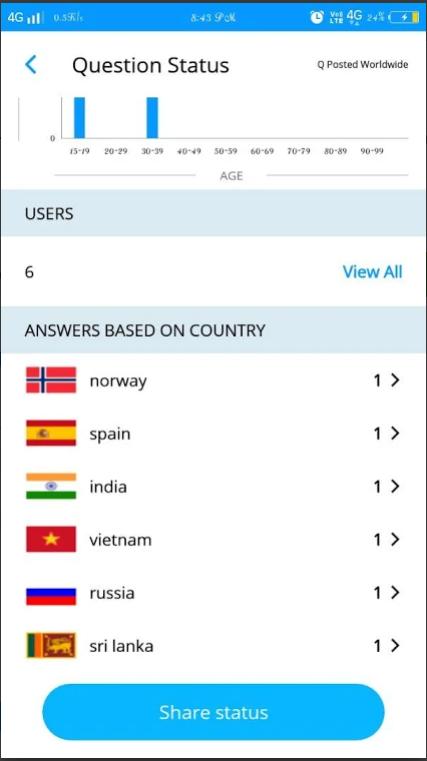This image is a screenshot from a cell phone display. At the top of the screen, there is a header labeled "Question Status," which is accompanied by a blue back arrow button on the left. Below this header, several cell phone status icons are visible.

Underneath the header, there is a bar chart with two prominent vertical blue bars. The bars represent age groups, with one bar marked at the "15 to 19" age range and the other at the "30 to 39" age range. The x-axis of the chart specifies "Age" in a gray font.

Beneath the chart, there is a light blue section labeled "Users" in black font on the left. Within this section, there is a white bar that displays the number "6." To the right of this white bar, it says "View All."

Further down, the screen indicates "Answers Based on Country," listing a total of six countries.